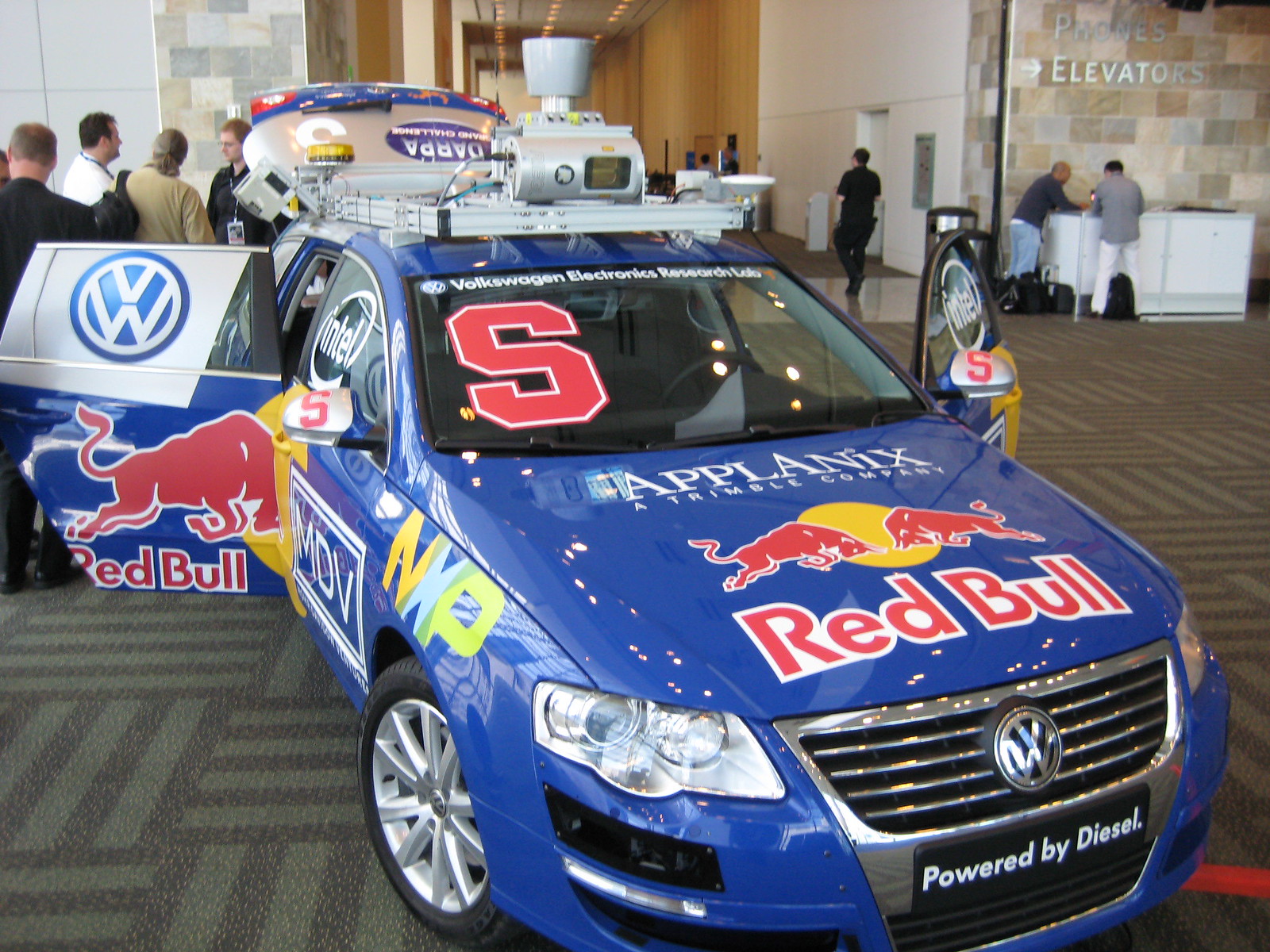In this indoor setting, the focus is on a prominently displayed blue Volkswagen sedan, heavily branded with Red Bull logos. The front of the vehicle features the Volkswagen emblem above a decal reading "Powered by Diesel." The car’s hood is adorned with several decals: in white text, it says "Applanix," followed by "A Trimble Company," and beneath these, the iconic Red Bull logo, consisting of a yellow circle with two red bulls charging at each other, accompanied by the text "Red Bull" in red with a white outline.

The windshield showcases additional branding, with the word "Volkswagen" across the top and a large red "S" with a white outline on the left side. The car is equipped with various pieces of mechanical or scientific equipment mounted on its roof, including a cylinder with attached piping.

The vehicle's back left and front right doors, as well as the trunk, are open, revealing that there is no one inside. Several individuals are gathered near the car, seemingly attentive to a speaker who is wearing an ID badge and a lanyard, possibly delivering a demonstration or discussion. 

In the immediate background to the right, there is a white desk with two people visible. Above them, a sign reads "Phone Elevator" in white text with an arrow pointing right. The area further back contains a hallway with tall, alternating white and brown wooden walls and a stone wall in the upper right corner featuring the word "Elevators" in a silver metal sign. The floor beneath the car is covered in a light and dark gray striped carpet.